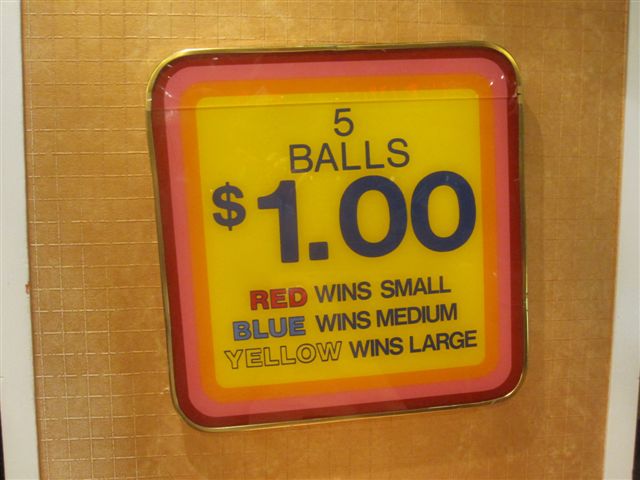This intricate image features a square with multiple layers and detailed text. Starting from the outermost layer, the square’s border is a striking metallic gold, followed by an inner border in dark red. Inside this dual-bordered frame are additional nested squares: a pink square, then an orange square, and finally, a yellow background that occupies about 60% of the remaining space.

Central to this composition, the text is arranged from top to bottom. The largest and most prominent text reads "Five Balls" in blue lettering, followed by a dollar sign and "1.00" directly underneath. Beneath this, smaller text provides game instructions: "Red wins small, Blue wins medium, Yellow wins large." The entire textual content is set against a light brown background with white edges, adding a neat and structured finish to the vibrant and playful design.